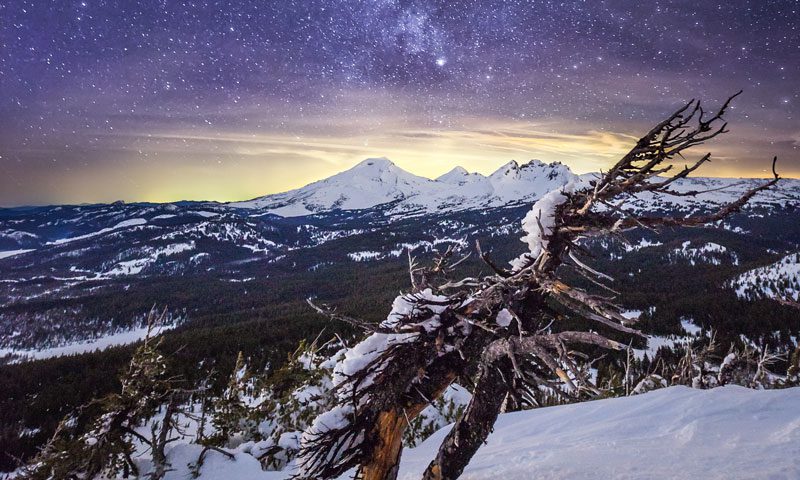The image depicts a striking winter landscape, characterized by a vast, snow-covered terrain. In the foreground, there are several dried-out tree trunks with their roots exposed, partially buried and accented with snow and ice. One prominently slanted tree appears windswept, missing several branches and strips of bark. The ground is thoroughly blanketed in snow, while patches of exposed land reveal dark green vegetation amidst the white expanse.

In the mid-ground, a dense pine forest stretches across the scene, with gaps exposing snow-covered ground between the trees. Further back, majestic snowcapped mountains with three distinct peaks dominate the horizon. The sky above is a captivating mix of silvery gold and purple hues, suggesting either dawn or dusk. The upper sky is dotted with twinkling stars, indicating a long exposure and adding a mystical quality to the tranquil, cold environment.